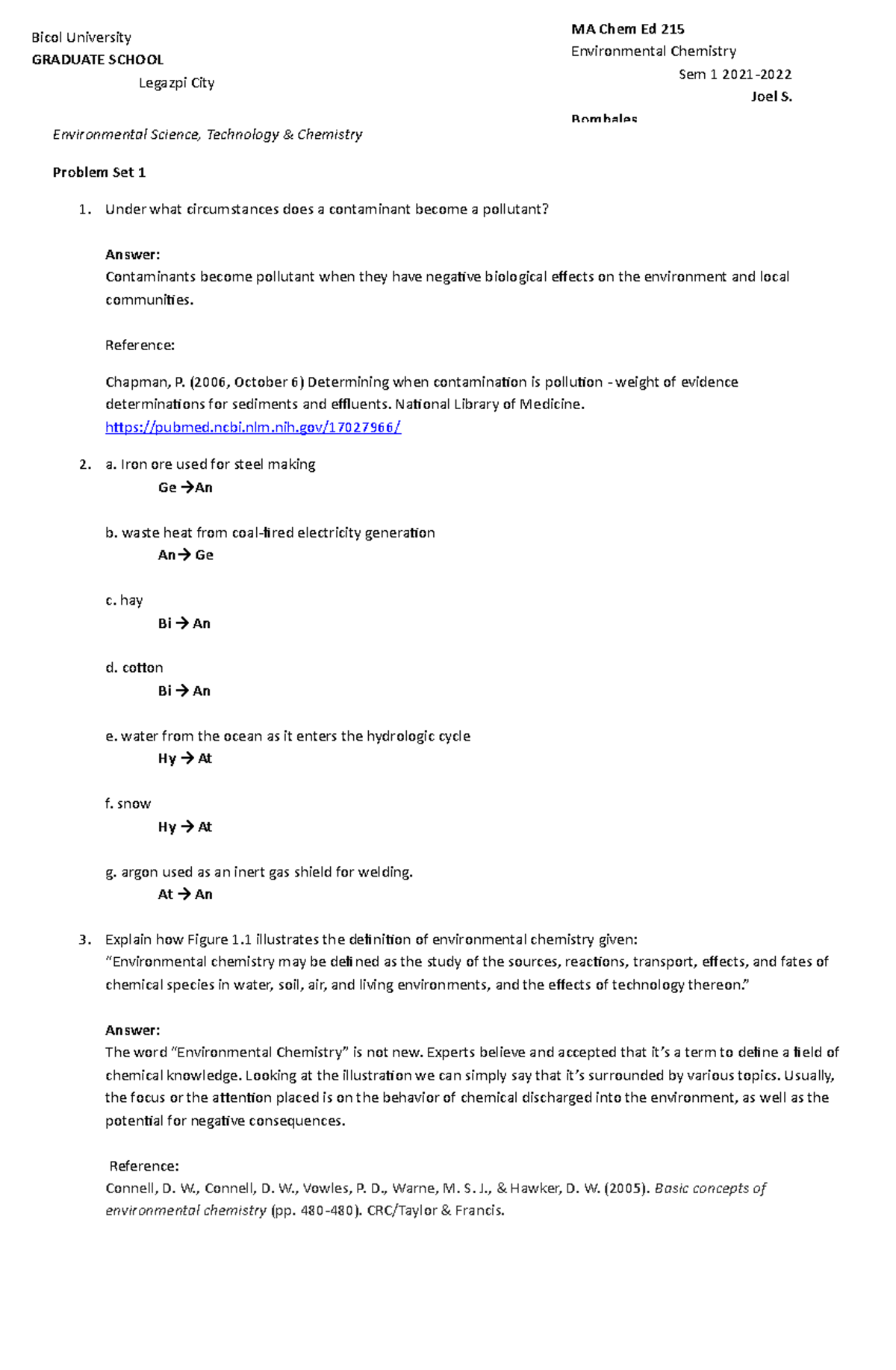This image is a screenshot of a test page from an exam. The background is white. In the upper left-hand corner, the text reads "Bicolle University," with the word "Graduate School" written beneath it. Further down, it mentions "Legazpi City." On the upper right-hand corner, the document specifies the course details: "M.A. Chem Ed 215, Environmental Chemistry," followed by "Semester 1 (S.E.M) 2021-2022." Below this, the name "Joel S." is noted.

Returning to the left side, the header reads "Environmental Science, Technology, and Chemistry." Directly below the header in bold font, it states "Problem Set 1." The problem description starts with “1,” and asks, "Under what circumstances does a contaminant become a pollutant?" The provided answer explains that "contaminants become pollutants when they have negative biological effects on the environment and local communities." The description continues in similar detail.